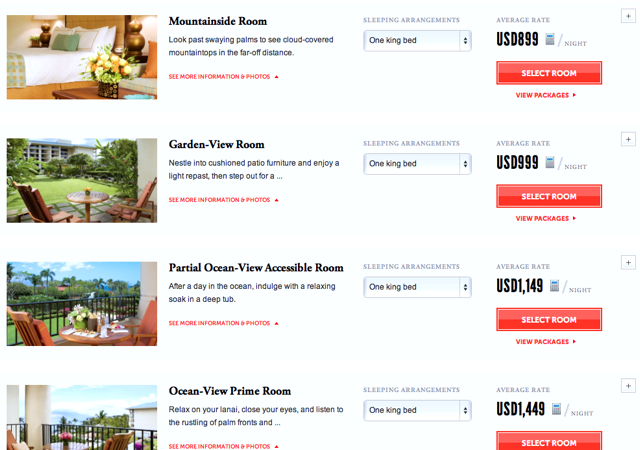The screenshot on the left-hand side of the screen showcases a selection of travel accommodations, including Airbnbs and hotels, available for travelers to browse. The first listing highlighted is a 'Mountainside Room' featuring a description: "Look past swaying palms and see cloud-covered mountaintops in the far-off distance." To explore further, there is red text reading "See more information and photos" accompanied by a clickable red arrow, which opens a dropdown menu with additional options.

Adjacent to this, a tab labeled 'Sleeping Arrangement' with an up-and-down arrow allows users to choose different bed configurations. The current selection shows "One King Bed." Another tab displays the average rate per night, listed as "USD 8.99/night," indicating that these rooms are on the more luxurious and higher-priced side. 

Additionally, another listing within the same interface features a 'Garden View Room' with a similar setup: "One King Bed" selected for the sleeping arrangement, priced at "USD 9.99/night." Users can explore various packages and room options on this website to find the perfect accommodation for their vacation.